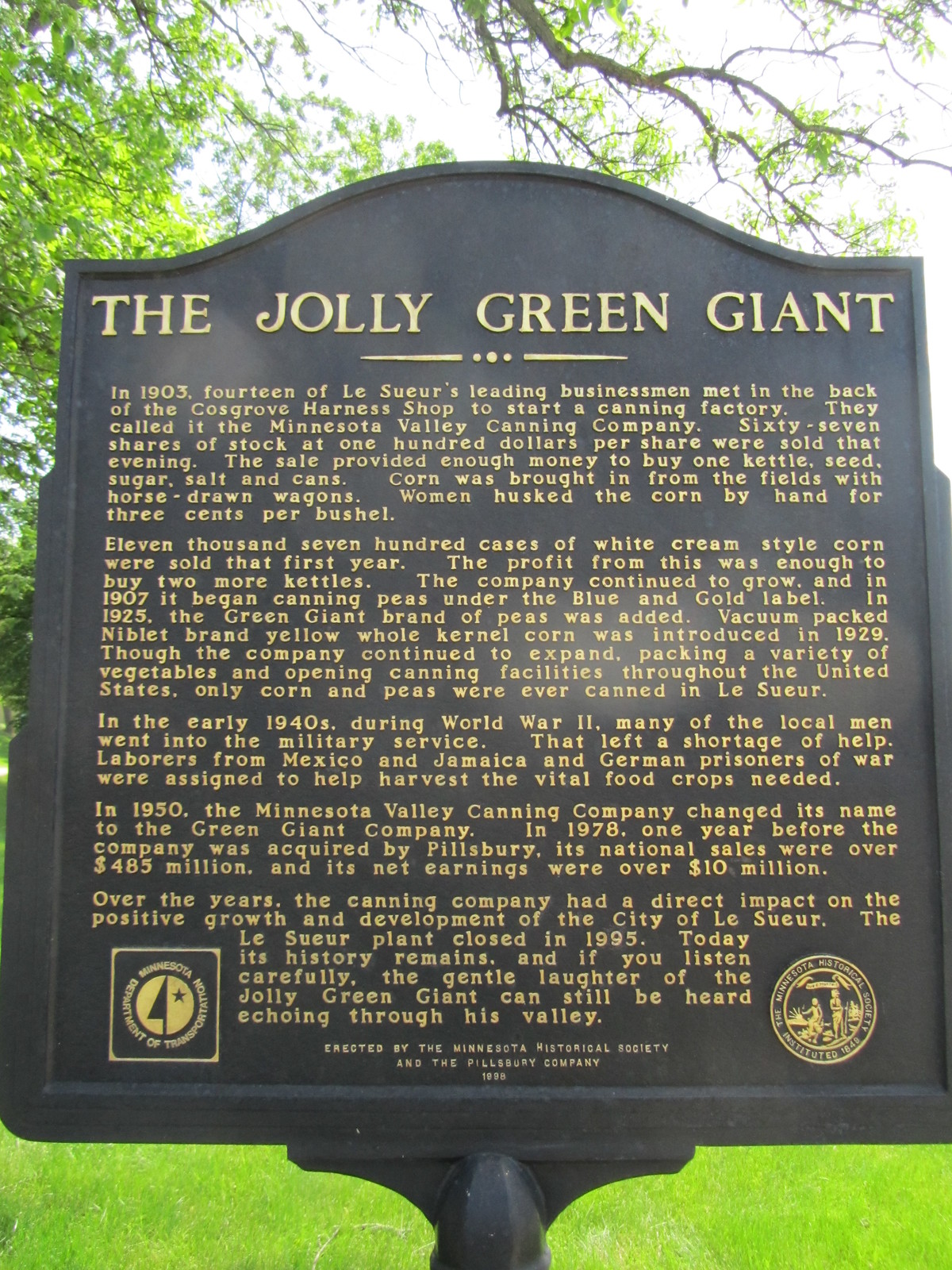The photograph captures an outdoor setting at a historical site featuring a detailed informative sign, likely erected by a state or government institution. The sign itself stands prominently in the center of the image and is crafted from metal with a dark gray or black background. The text is inscribed in gold or silver font and meticulously chronicles the origins of the Green Giant brand.

The narrative on the sign begins with "The Jolly Green Giant" and recounts the formation of the Minnesota Valley Canning Company in 1903 by fourteen leading businessmen of LeSeul. They convened in the back of Cosgrove Harness Shoppe to establish the venture, selling sixty-seven shares of stock at $100 each to raise funds for essential supplies. Initial efforts involved harvesting corn with horse-drawn wagons, women husking the corn by hand for three cents per bushel, and selling 11,700 cases of white cream-style corn in their first year.

The company's growth is further detailed, noting the beginning of pea canning under a blue and gold label in 1907 and the introduction of the Green Giant brand in 1925. Significant innovations include the debut of vacuum-packed Niblet brand yellow whole kernel corn in 1929. Despite expanding its operations throughout the United States, the LeSeul facility exclusively canned corn and peas.

The historical account continues into the early 1940s, describing how World War II led to labor shortages filled by workers from Mexico, Jamaica, and German prisoners of war. The company rebranded as the Green Giant Company in 1950 and achieved substantial financial success by 1978, just before being acquired by Pillsbury, with national sales exceeding $485 million and net earnings over $10 million.

The text concludes by highlighting the significant impact of the canning company on LeSeul's development and its eventual closure in 1995. There's a poetic note indicating that the legacy of the Green Giant endures, symbolized by the mythical laughter of the Jolly Green Giant echoing through the valley.

The background of the photograph features a vibrant, sunny day with a lush, green forest comprising trees and grass. The sky is clear, complementing the earthy tones of green, brown, gray, gold, and black present in the image. Multiple logos, possibly of the Minnesota Historical Society and the Pillsbury Company, adorn the sign's left and right sides but are too small to read clearly. The image, shaped as a vertical rectangle, shows the signpost and its surrounding natural habitat, capturing the essence of the historical monument.